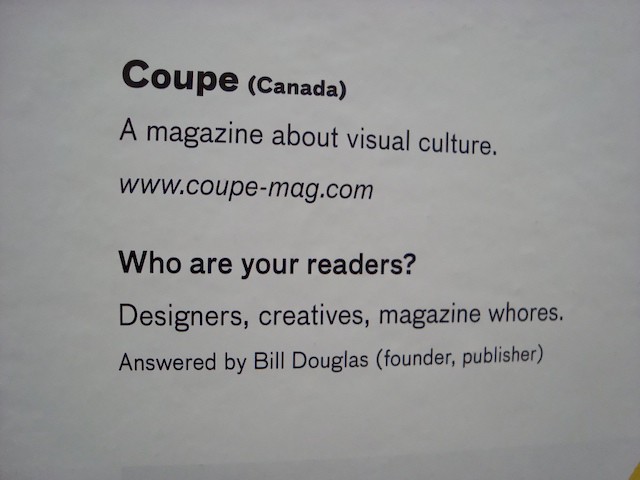The image appears to be a page from a magazine titled "Coop Canada," which is focused on visual culture. The page features black text on a white background, prominently displaying the magazine's name, "Coop [Canada]," in bold. Below it, a line in regular font explains that it is "a magazine about visual culture," followed by the website "www.coop.com," written in italics. A noticeable gap divides this section from the next, which poses the question, "Who are your readers?" This line is slightly bolder than the others. It is followed by potential reader categories: "Designers? Creatives? Magazine whores?" The answer, provided by "Bill Douglas, [founder, publisher]" also appears on the page. In the bottom right corner, there's a hint of an orangish color, likely part of an off-screen image, suggesting this could be the introductory page meant to engage and identify the magazine's target audience.